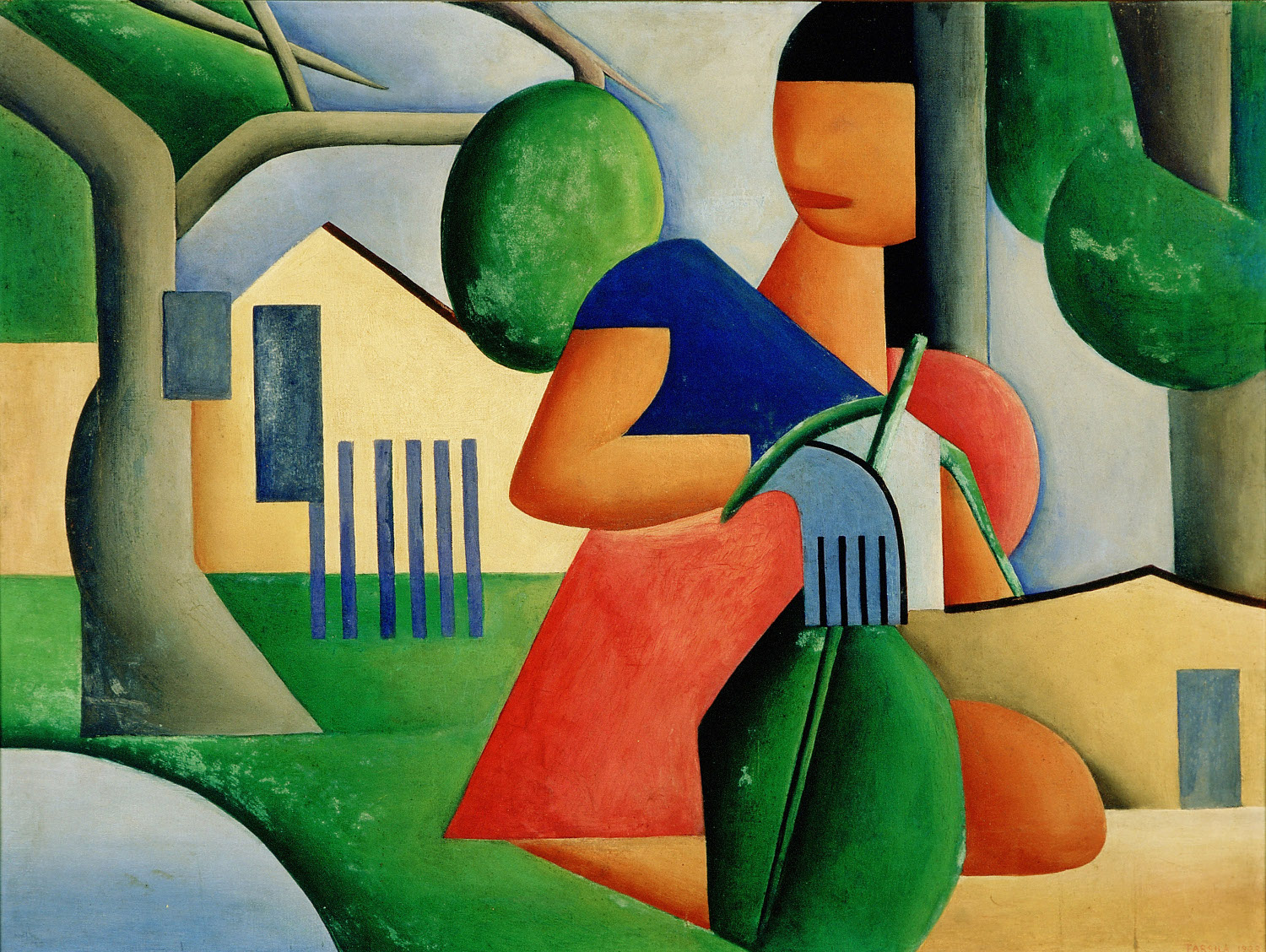This abstract, Impressionist-style image features a vibrant palette of bold primary colors and geometric shapes, reminiscent of Picasso's work. Dominating the center is a depiction of a woman, characterized by blocky, angular forms. Her black hair with pronounced bangs frames her faceless head, save for a distinct red shape representing her lips. She is presented in a kneeling position, clothed in a short-sleeve blue shirt, a red section likely representing the rest of her shirt, and bare knees touching the brown ground. Her right hand, donned in a light blue glove, clutches a large green leaf, suggesting she is gardening.

Surrounding her are snippets of an outdoor setting: green grass, a narrow blue fence, and a blocky tree with multiple branches, all contributing to the image's dynamic composition. A distant house with abstract, block-like windows and possibly another building to the right evoke a sense of depth and environment. A semi-circle in the lower left corner symbolizes a light blue lake, enhancing the picturesque scenery. Despite the absence of a signature, the painting's rich color scheme and well-executed geometric shapes speak volumes about the artist's skill.